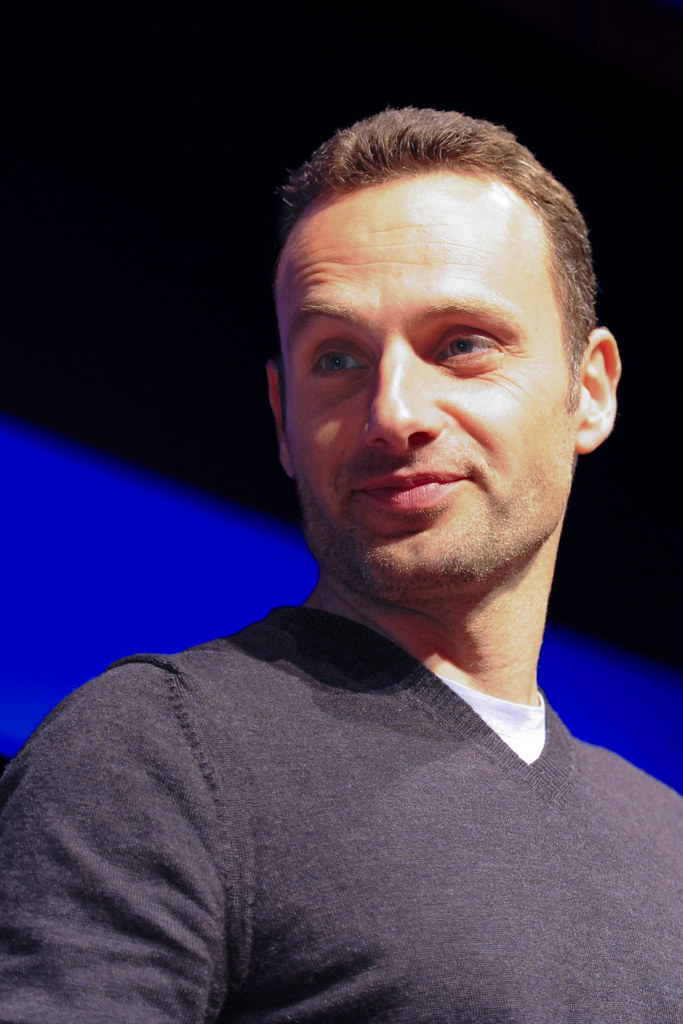This is a high-resolution color photograph of a white male with light skin, resembling actor Andrew Lincoln from "The Walking Dead." The image captures him from the top of his chest to his head. He has short, dark hair with some stubble and bluish-green eyes. He is wearing a dark gray, long-sleeve v-neck sweater over a white t-shirt. The man has a slightly raised right eyebrow and a smirk on his face. He is looking to his right, not directly at the camera. The background features a sharp contrast with a black upper section and a bright blue stripe or section below it. The image is bright and clear with no additional text or people.